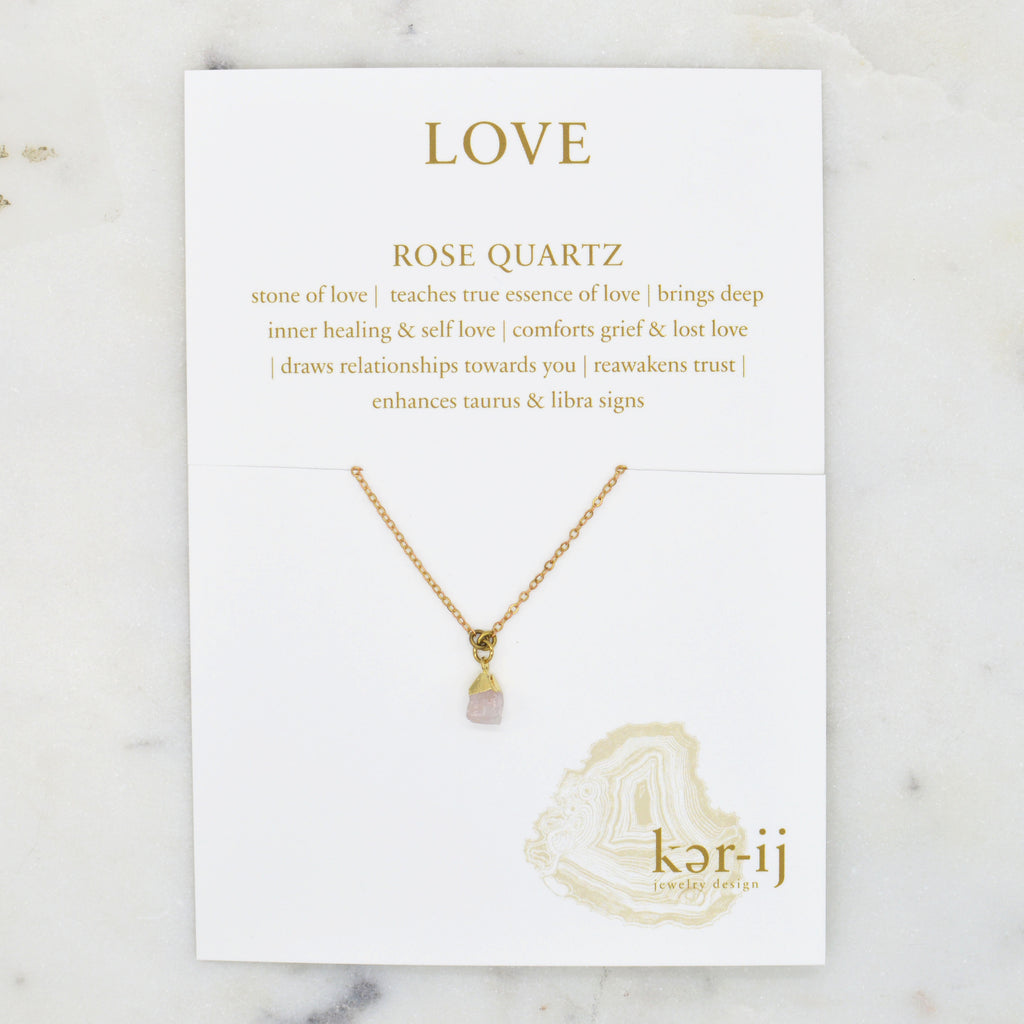The image showcases a delicate gold chain necklace elegantly displayed on a white rectangular card, likely made of poster board material, positioned on a white marble surface accented with natural gray and gold veining. The necklace features a small, lavender-colored rose quartz stone as its charm. The front of the card is emblazoned at the top with the word LOVE in capitalized, gold letters, followed by ROSE QUARTZ in a slightly smaller, bold font. Below that, in a more diminutive, lowercase font, the card reads "stone of love, teaches true essence of love, brings deep inner healing and self-love, comforts grief and lost love, draws relationships towards you, reawakens trust, enhances Taurus and Libra signs." The back part of the necklace, along with its clasp, is hidden behind the card, accentuating the charm and the inscriptions. Additionally, a gold stamp that reads CARE EACH appears in the lower right corner of the card, enhancing its luxurious presentation.